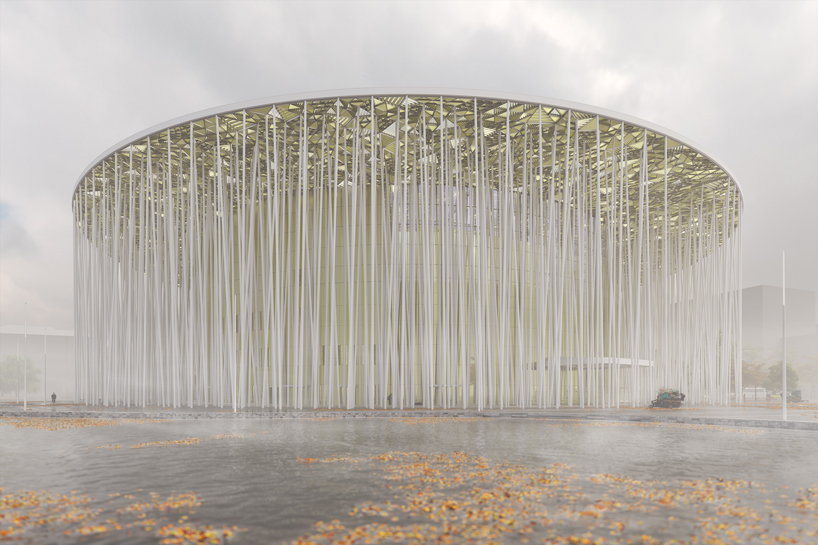The image captures a massive and architecturally unique circular building with a flat roof, accentuated by white columns that encompass its exterior. The underside of the roof features intricate golden triangular designs connected by radiating lines, adding a touch of elegance. The building overlooks a large, gray pool of water adorned with brown leaves, giving the scene a serene and slightly foggy ambiance. The water's edge is framed by a flat, gray surface. Underneath the roof, the interior is characterized by greenish-yellow tinted glass, creating a wider ceiling effect. Suspended from the ceiling are multiple white threads or strings, descending like delicate droplets, enhancing the building's majestic and somewhat mysterious appearance. The entire scene is set against a backdrop of hazy, cloudy skies, with a small person visible on the left, highlighting the structure's grand scale and beauty.